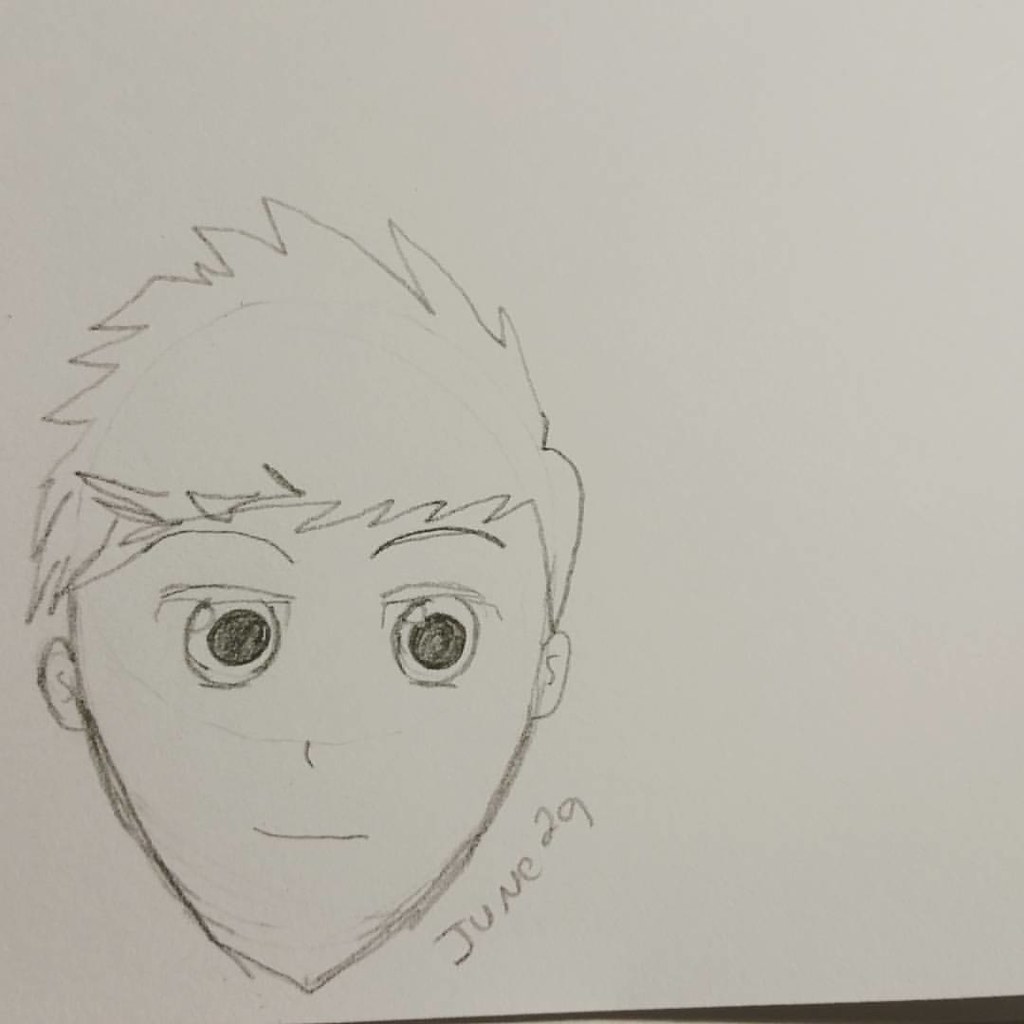This detailed caption offers a vivid description of the image:

A charcoal drawing on a white square paper depicts the face of a young boy. The square paper is slightly lifted, revealing a thin black background at the bottom left corner and a diagonal line narrowing towards the center, creating an off-center, left-side composition. The boy’s face features messy, spiky hair, with similarly spiky bangs hanging over his forehead. His thin-lined eyebrows rest above large black pupils, giving an intense gaze. Below, his nose is represented by a simple half-moon line, and his mouth is a thin horizontal stroke. His face tapers into a pointy chin, framed by small ears on either side. The date, "June 29th," is inscribed to the right of his chin, near the bottom of the drawing.